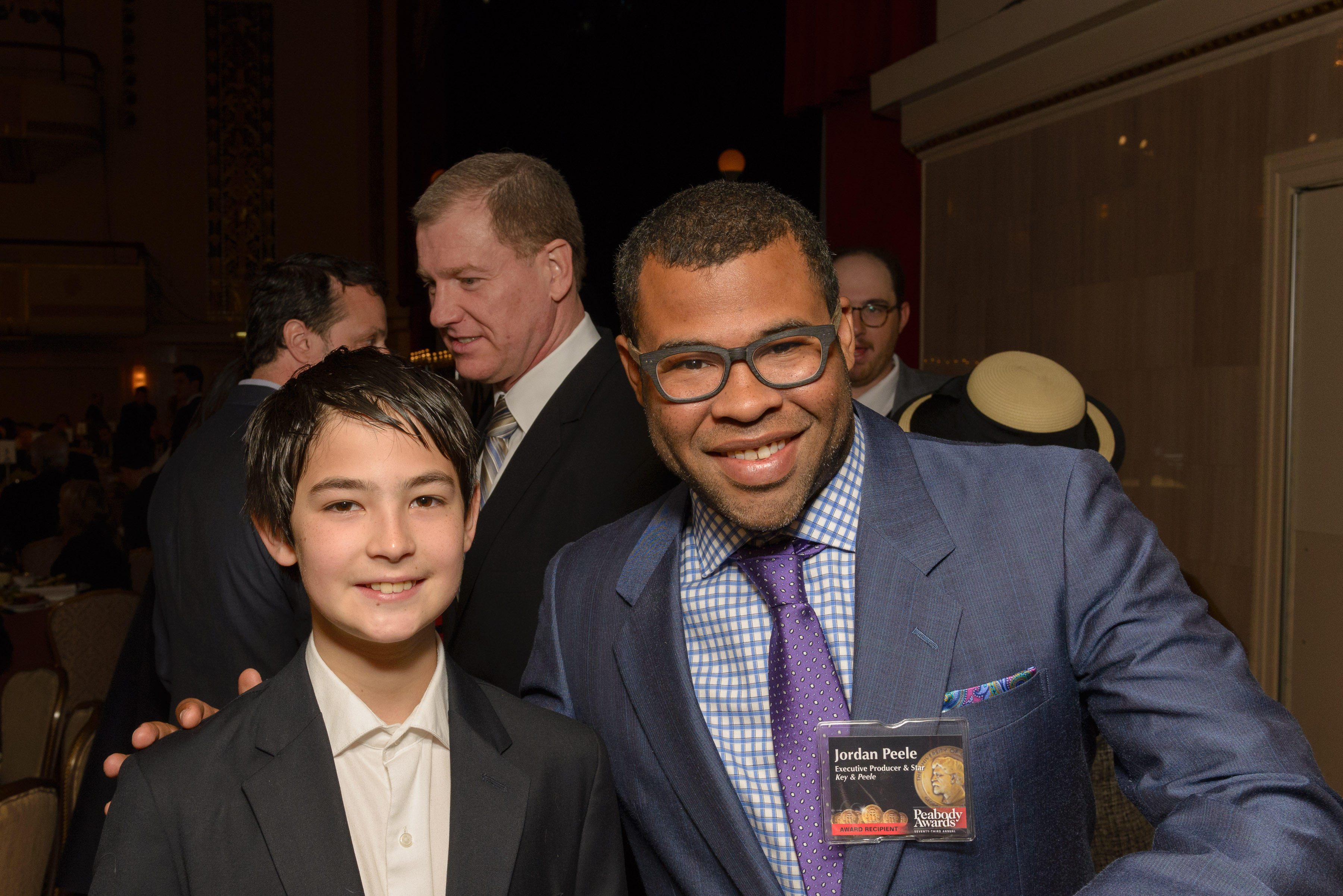The photograph captures Jordan Peele, the renowned comedian and executive producer known from the "Key and Peele" show, posing with a young boy. Jordan Peele, identifiable by his name tag that reads "Jordan Peele, executive producer and star, Key and Peele, award recipient, Peabody Awards," is wearing a navy blue suit jacket, a blue and white checkered shirt, and a purple tie. He has short black hair, glasses, and a smile on his face. The young boy beside him, who appears to be around 9-10 years old, is dressed in a black suit jacket over a white collared shirt, and has short brown hair. They are standing in what seems to be a large gathering or awards ceremony, as evidenced by the chairs and tables in the background. The setting is indoors with brown walls and a door, filled with people also dressed formally, likely attending the same event.